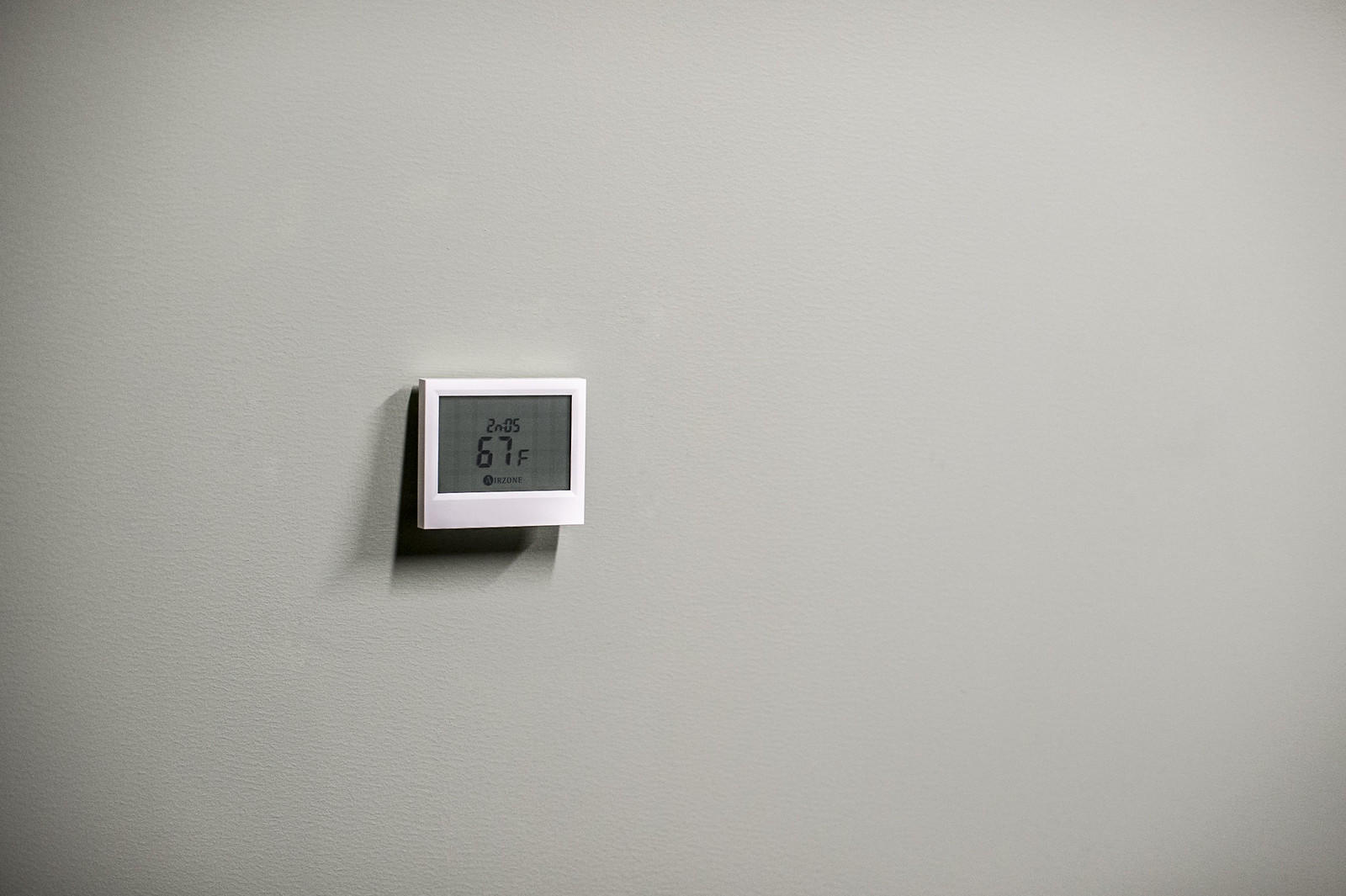The image captures a white, textured wall adorned with a digital thermostat positioned on the left side. The wall's surface displays a rough, raised texture in certain areas. Surrounding the entire frame of the image, there's a vignette effect created by a dark, blackish-gray shadow. This shadow is most prominent in the top left corner, extends down the left edge, and intensifies again in the bottom left corner before stretching towards the bottom right. A faint shadow continues along the right side, tapering off to a subtle hint of grayish-black at the top right corner.

The digital thermostat, encased in a white frame, prominently displays a grayscale screen. On the screen, black numbers read '2n05' alongside the temperature '67°F'. Below the temperature, additional text in black is visible. The thermostat itself is square-shaped and contrasts starkly against the textured white wall.